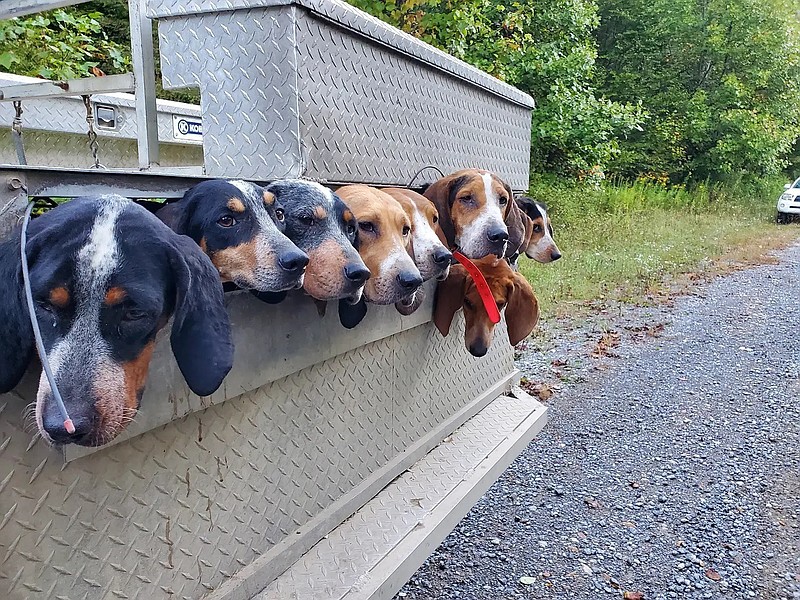This outdoor, daytime photograph captures the back of a silver-metal work truck parked on a gravel road amidst wooded surroundings. Prominently featured in the back are the heads and floppy ears of eight dogs, likely Beagles or Basset Hounds, in various shades of dark, light brown, and dark brown muzzles. Their faces peek out from a metal casing, suggesting some transportation or containment system, possibly for securing the dogs. To the upper right of the image, partially visible, is the bumper of a small white car. The background is filled with grass, trees, and brush, emphasizing the rugged, unpaved setting.